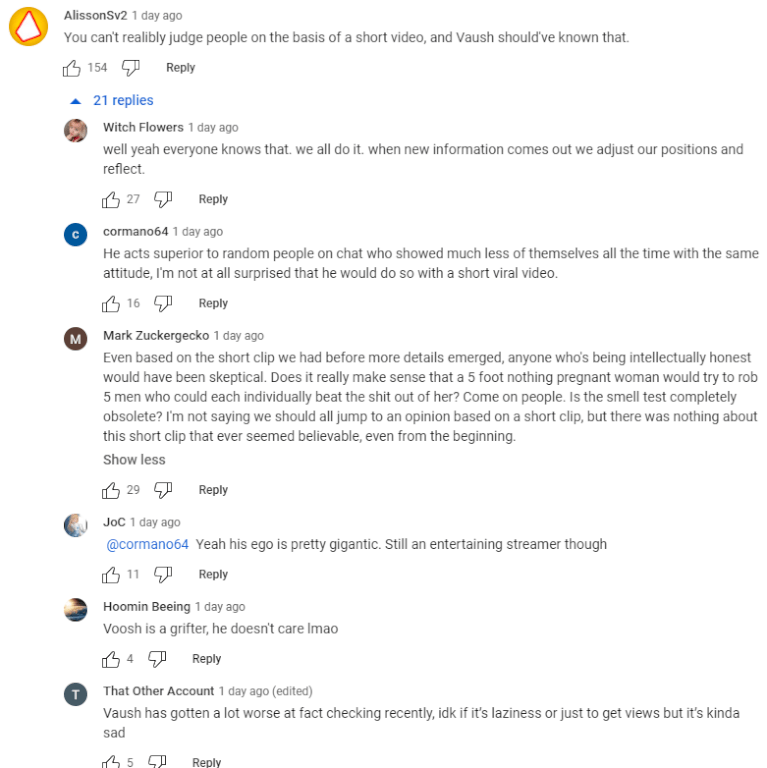Certainly! Here is a detailed and cleaned-up descriptive caption:

---

The image is a screenshot of a YouTube comments section, featuring a total of seven comments from various users. Each comment is displayed with the commenter’s profile picture, username, the time it was posted, thumbs up and thumbs down buttons, and a reply button. 

1. The first comment criticizes the notion of judging people based on short video clips, stating that "you can't reliably judge people on the basis of a short video, and Vau should have known that."
2. The second commenter agrees, indicating that it's common knowledge and that people update their opinions as new information becomes available: "well yeah, everyone knows that, we all do it, when new information comes out, we adjust our positions and reflect."
3. The third comment criticizes a person for acting superior in chat and mentions skepticism about a widely circulated short video: "he acts superior to random people in chat, shows much less of themselves all the time, and the same attitude, I'm not all that surprised he would do so with short viral video. Even based on the short clip we had before details emerged, anyone who's being intellectually honest would have been skeptical, it doesn't really make sense that a 5 foot nothing pregnant woman would try to rob 5 men who could each individually beat the shit out of her."

The comments continue in a somewhat chaotic manner, typical for a YouTube comments section. The background is plain white, and the overall layout and colors are characteristic of YouTube’s interface, with clickable text appearing in blue. Other than those elements, the display follows YouTube’s standard design with no additional colors or hidden details.

---

This rephrased caption adheres closely to the original content while enhancing readability and providing a comprehensive description.